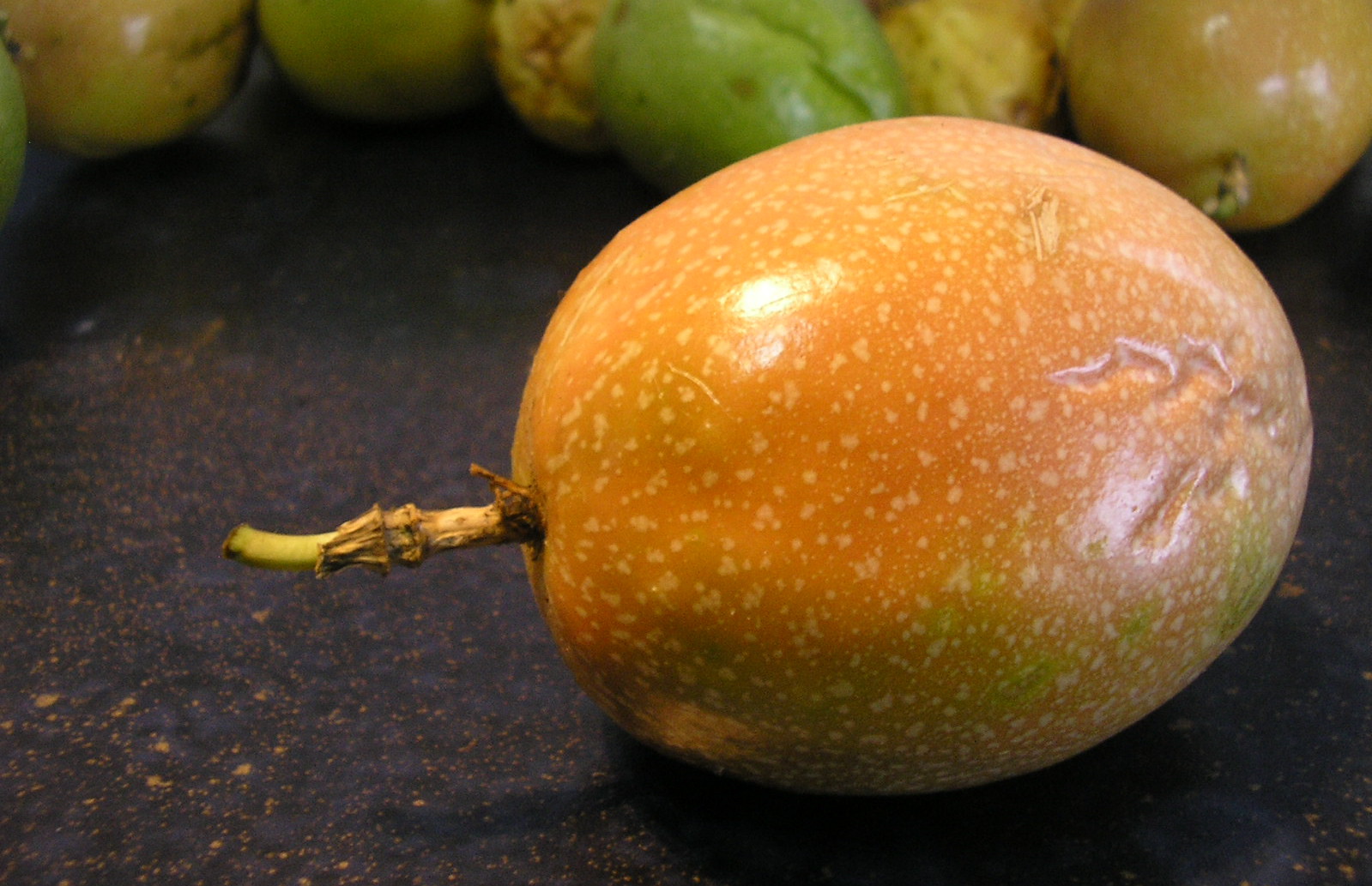This close-up image showcases a vibrant assortment of fruit arranged on a surface that appears to be a black table with small gold flecks. Dominating the foreground is an oval-shaped, orange-colored fruit, likely a papaya, with a brown stem that transitions to green at the tip. The papaya's skin is dotted with tan-colored spots and exhibits some pink gouge marks that seem superficial. The fruit's shiny surface reflects light, revealing some white and green blemishes, potentially indicating mild bruising or damage. In the background, a row of various fruits is visible, including green and yellow pears with brown spots, and possibly some apples. The green pears appear firm while the yellow pears suggest they might be softer. The fruits in the backdrop create a visually appealing contrast with the prominently featured papaya in the foreground.